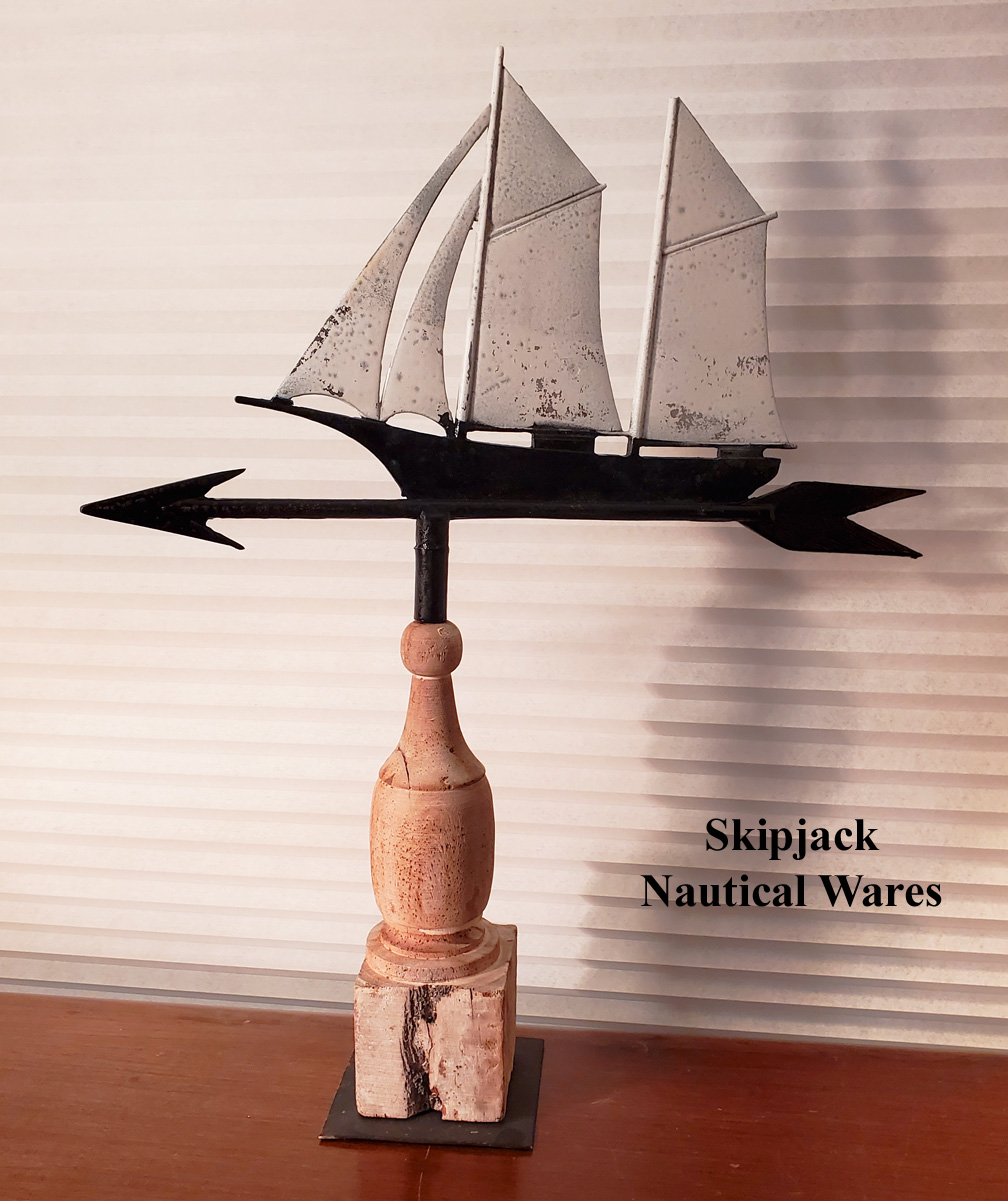The photograph showcases an ornamental piece meticulously placed on a medium brown wooden desk before a set of white horizontal blinds. To the right of this piece, the words "Skipjack Nautical Wares" are distinctly visible in black. The ornamental object itself is anchored on a square black metal base, which supports a natural wooden block. Emerging from this base is a wooden post reminiscent of a bedpost or a railing, topped with a black metal arrow pointing to the left. Resting on this arrow is a distressed black ship, complete with three white sails marked with scattered black dots, crafted to evoke an aged, vintage aesthetic. The piece intricately combines wood and metal elements, creating a visually striking and thoughtfully designed nautical-themed décor item.